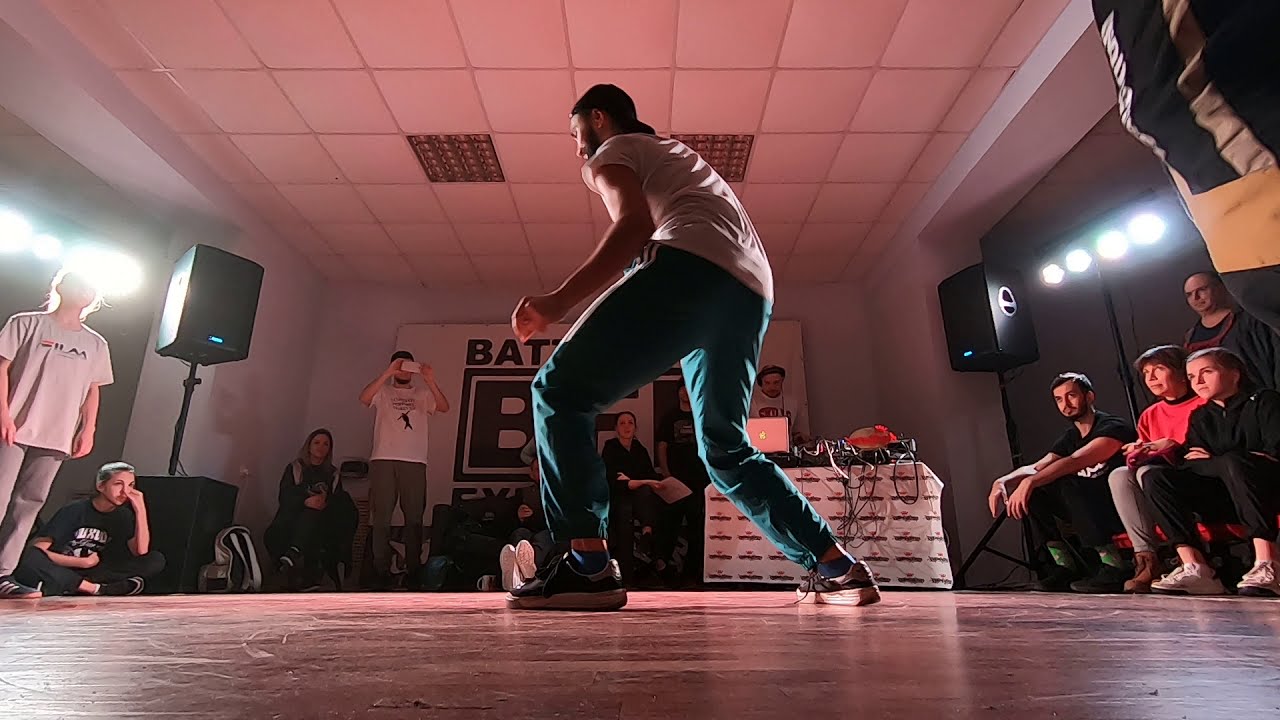This photograph features an indoor dance studio with light brown wooden floors, somewhat glossy yet marked with scratches, and a ceiling of white square tiles. The main subject is a male dancer in the center, captured in mid-move, bent over with his left leg extended forward. He is wearing a white t-shirt and blue pants with black and white shoes. The walls are painted gray and decorated with a large sign at the back displaying the letters "B.A.T."

The room is filled with spectators, some standing and others sitting around the edges. To the dancer's right, three people are seated watching him, with a standing man behind them. To their left, a table cluttered with wires and possibly a laptop sits near a tall speaker reaching up toward the ceiling.

In the left-hand side of the image, several people are seated, some on couches, observing the dancer. One person is taking a picture with a cell phone, dressed in a white t-shirt and greenish pants. Next to him, a woman is sitting with her legs crossed. Another large speaker stands near them. A girl in a black t-shirt sits on the floor with her hand near her face, partially obscured by light, while another girl sits beside her facing away from the camera. The setup, complete with a DJ table at the front and sound systems scattered around, suggests a dance competition environment.